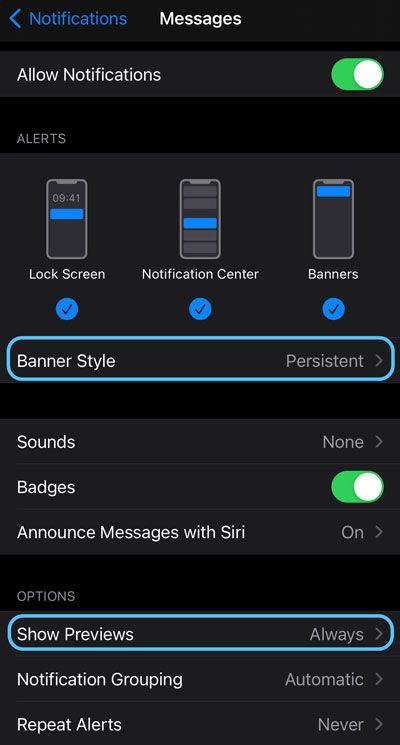This image is a screenshot of a settings menu on a mobile phone. At the top, there is a black bar featuring the word "Notifications" in purple font, alongside a small purple arrow pointing left. To the immediate right in the center, "Messages" is displayed in white font. Below this header, there is a gray rectangle containing the text "Allow Notifications" in white, accompanied by a green toggle switch that is currently turned on.

Underneath, there is a black rectangle with the word "Alerts" in gray font. Following this section, another gray rectangle presents three images of smartphones aligned horizontally. Each image is labeled: "Lock Screen" on the left, "Notification Center" in the middle, and "Banners" on the right. All three options are marked with a blue check.

Further down, there is an option labeled "Banner Style," set to "Persistent," which is circled in blue. Beneath this, several options are listed: "Sounds," which is set to "None"; "Badges," with a green toggle indicating it is turned on; and "Announce Messages with Siri," which is set to "On." Finally, at the bottom, there is a section titled "Options," where "Show Previews" is set to "Always," and this option is also circled in blue.